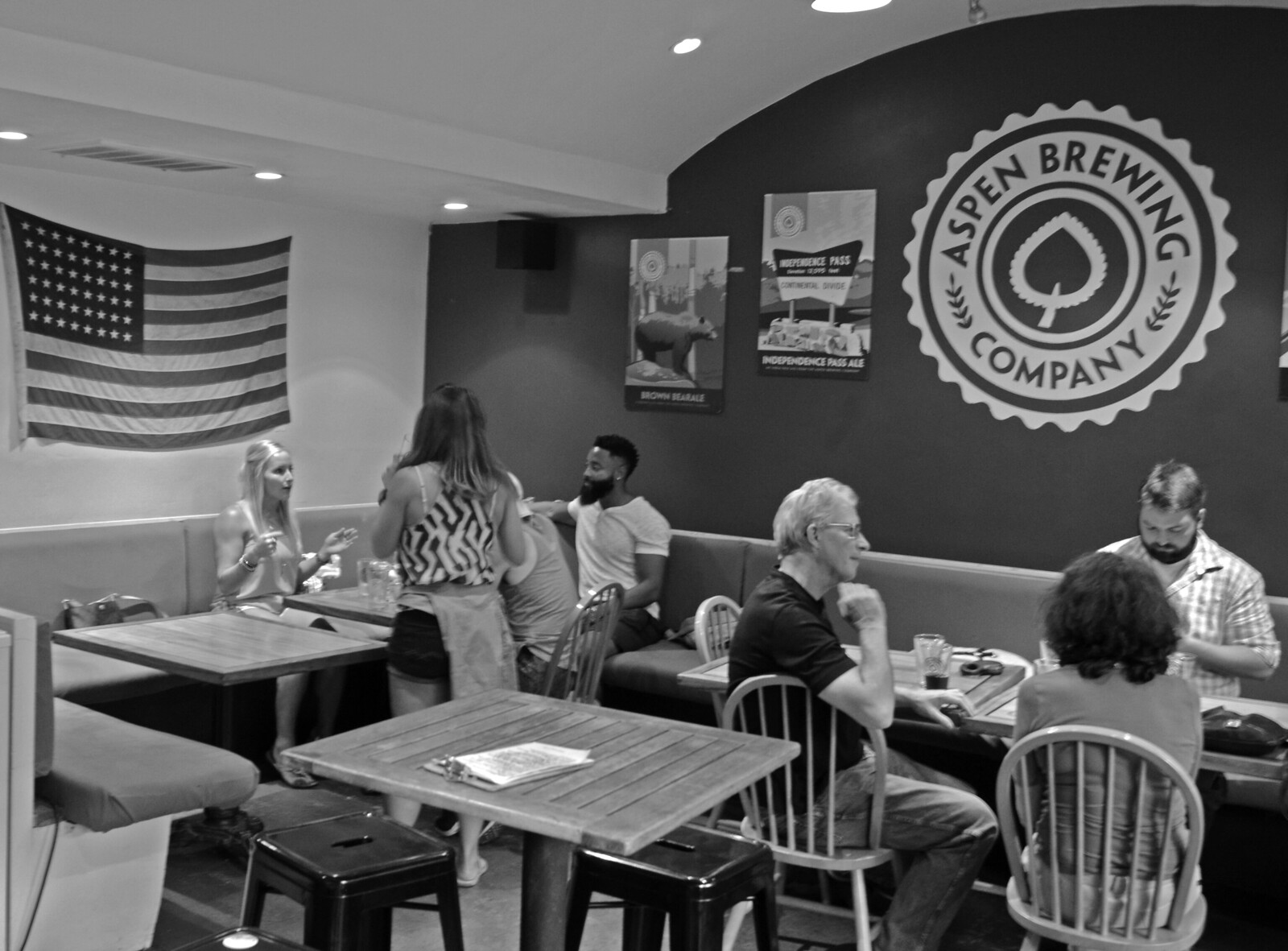In this black and white photograph of what appears to be a restaurant or cafe, the interior is detailed and thoughtfully arranged. The space features tables and chairs scattered throughout, with some tables occupied and others empty. Along the walls, there are booth-style tables with attached benches. The back wall, a darker shade contrasting with the white-painted left wall and ceiling, prominently displays a large circular logo of "Aspen Brewing Company" adorned with a wheel spoke design and a flower in the center. Under this logo, a few indistinct pictures can be seen.

On the left wall, an American flag is prominently displayed. Here, a group is seated comprising an older man in a dark polo shirt, a middle-aged man, and the back of a woman with dark hair. Adjacent to this group is a table where a young blonde woman in a white blouse, a seated dark-skinned man in a white t-shirt and black pants, and another barely visible individual are engaged in conversation. Standing nearby appears to be a waitress, identifiable by her apron, attending to the patrons. The waitress, with brunette hair, has her back towards us. Additionally, there are two empty tables in the foreground that further suggest the bustling yet unoccupied parts of the room, reflecting a moment in time within this cozy dining establishment.